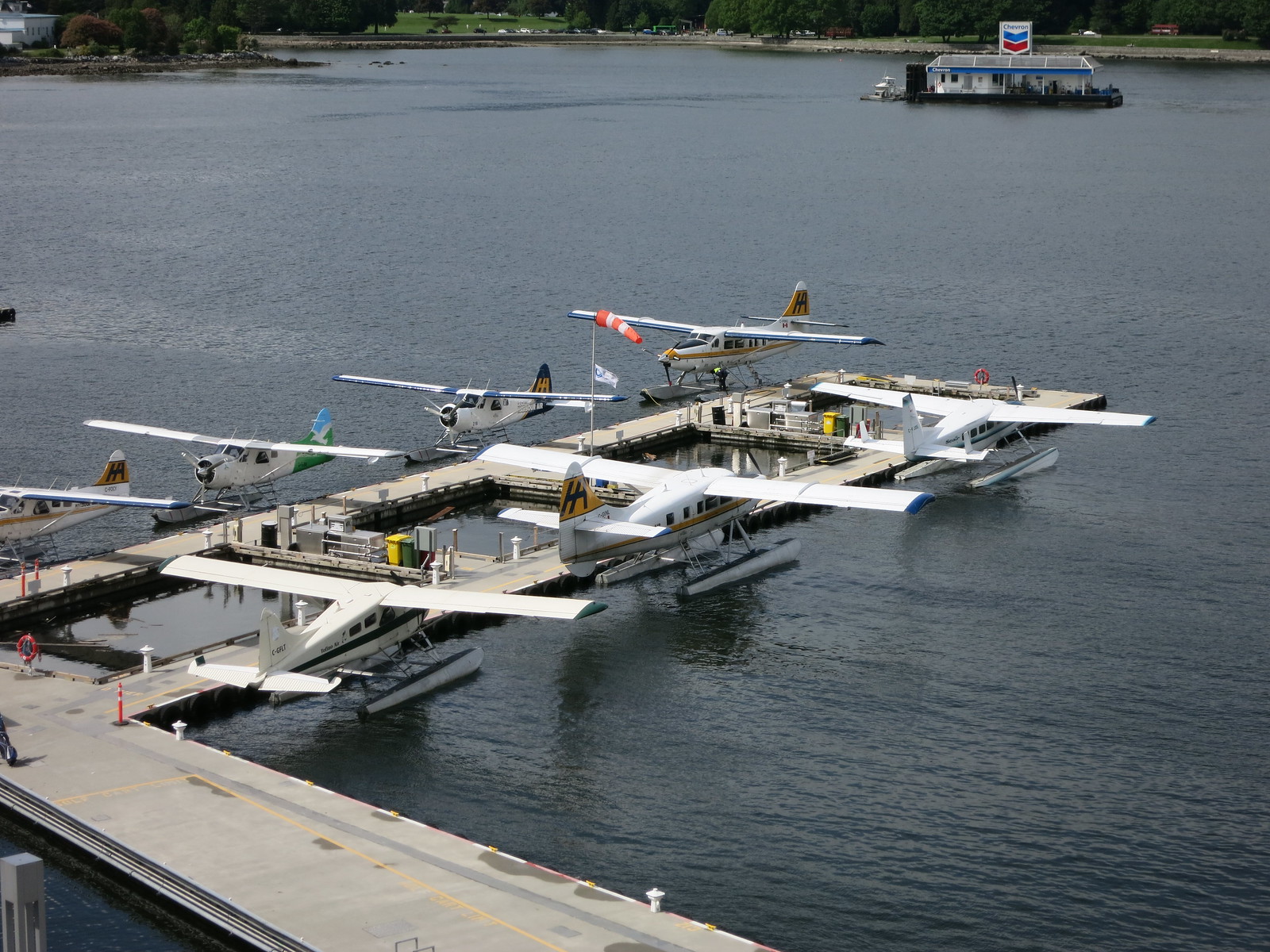This is a color, daytime photograph capturing a serene lake scene featuring a small, plain dock and a man-made pier that extends from the bottom left to the middle right of the image. Moored along the dock are seven single-engine airplanes, equipped with flotation devices for water takeoffs and landings. The planes, primarily white, are arranged in two rows: four face towards the bottom left and the camera, while three face away towards the right. Each plane features distinctive stripes in blue, yellow, and green.

The background showcases the calm, still waters of the lake, reflecting the sunny day. Prominently, a floating Chevron gas station with its signature Chevron sign—displaying the bold blue, white, and red colors—sits on a small island in the middle of the lake. The gas station includes a white building with blue trim. A cement road leads to the dock, extending out into the water. Further in the background, there is a sandy beach and a thin green landscape, adding to the tranquil atmosphere. There are no people visible in the scene, emphasizing the quiet solitude of this picturesque lakeside setting.